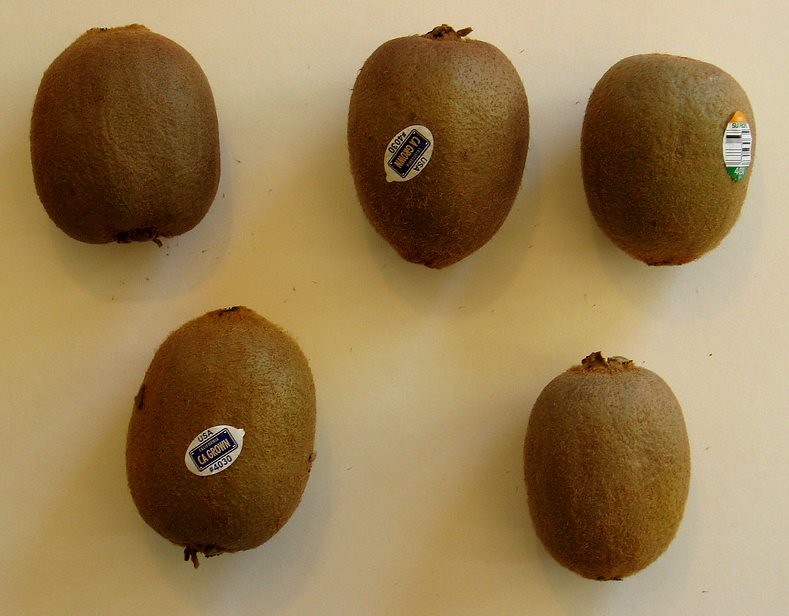This is a detailed photograph of five healthy kiwifruit placed on a white surface, seemingly fresh from the store. Three of the kiwis feature produce stickers with a distinctive design: a blue and white background resembling a California license plate, adorned with the text "CA Grown" and "USA" in blue, along with the number "4030" in white font. One of these stickers is positioned upside down. Another kiwi has a different sticker that showcases a mix of green, white, black, and orange colors, though the text on it is not entirely legible. The kiwifruit are arranged in a neat layout, with three on top and two at the bottom, creating a visually pleasing composition. They are brown and fuzzy, showing no signs of blemishes, and are lit by a subtle golden light that enhances their color.